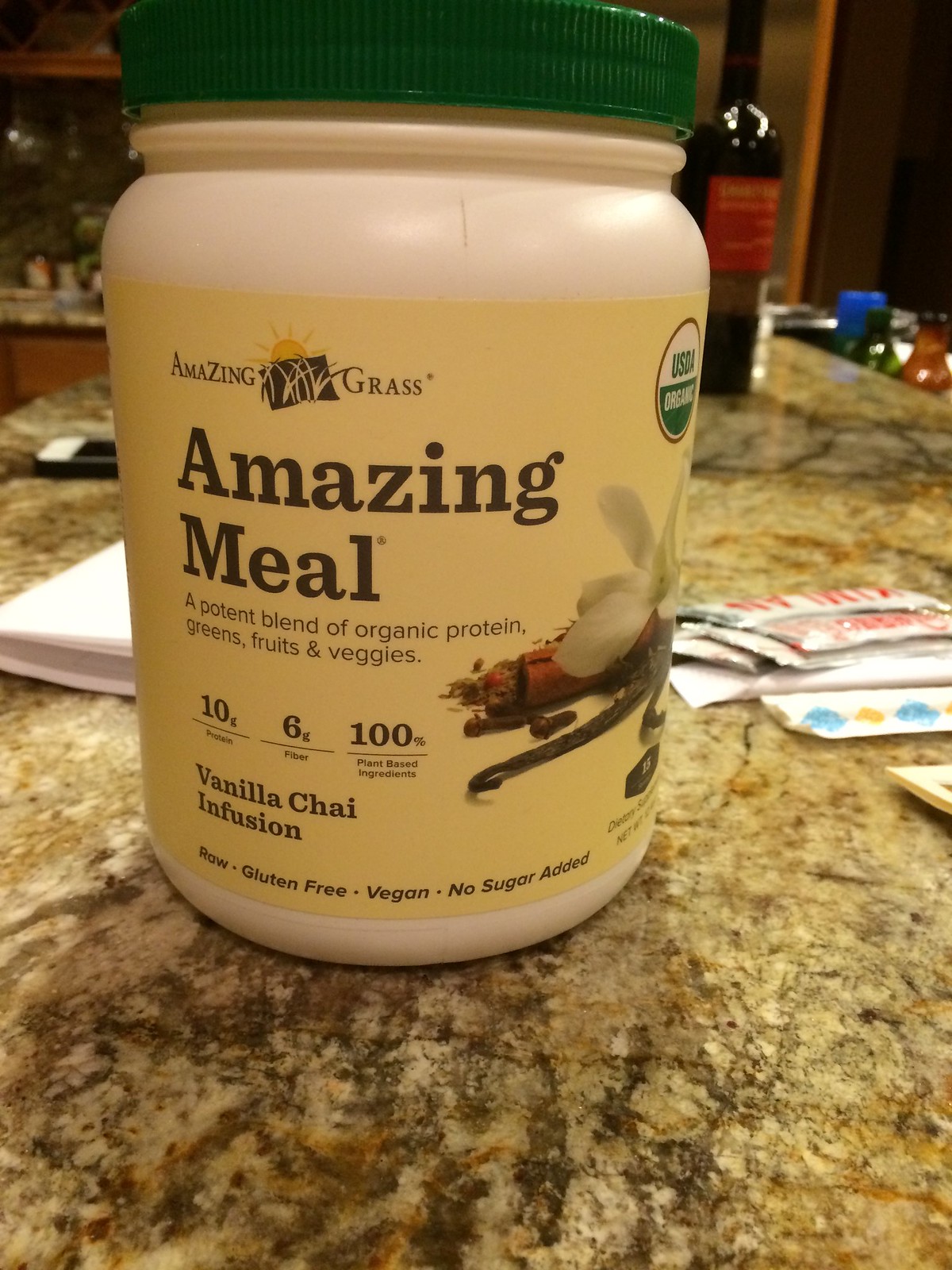The photograph captures a cozy kitchen setting, focusing on a kitchen counter made from stunning granite or quartz, characterized by a vibrant yellow base interspersed with brown, green, and neutral tones forming a unique, random pattern. Various everyday items are scattered across the counter, including a cell phone and an assortment of packets—possibly soy sauce packets—alongside a mysterious white object. Dominating the scene is a large plastic container with an off-white body and a green lid, centrally placed. The container features a vibrant yellow label emblazoned with the text "Amazing Grass, Amazing Meal," promoting a potent blend of organic protein, greens, fruits, and vegetables. The label details that the product offers 10 grams of protein, 6 grams of fiber, and is composed entirely of 100% plant-based ingredients, specifically noted as being a vanilla chai infusion. Additionally, it boasts raw, gluten-free, vegan characteristics with no added sugar, and partial images of ingredients adorn the label. A wine bottle is also visible on the counter with more kitchen paraphernalia subtly receding into the background, adding to the homely vibe of the image.